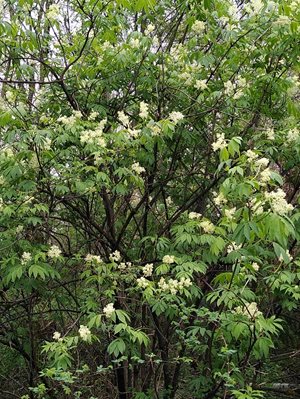This photograph captures a richly detailed outdoor scene during the day, dominated by a variety of lush trees and possibly some large bushes, all covered with bright green leaves. The branches of these trees are dark, almost blackish-brown, and adorned with numerous flowers that are cream to white in color. The leaves vary slightly in shades of green and light yellow, adding depth to the vibrant foliage. Despite a few branches lacking leaves, the verdant growth is thriving, suggesting ample rainfall. The sky behind the trees is a bright, cloudy white, indicating an overcast day. This scenic snapshot, taken from a low angle, shows the trees ascending from short in the foreground to taller heights, completely framing the picture within its rectangular shape. The scene, possibly set in a park, exudes tranquility and the robust vitality of a well-watered natural habitat.